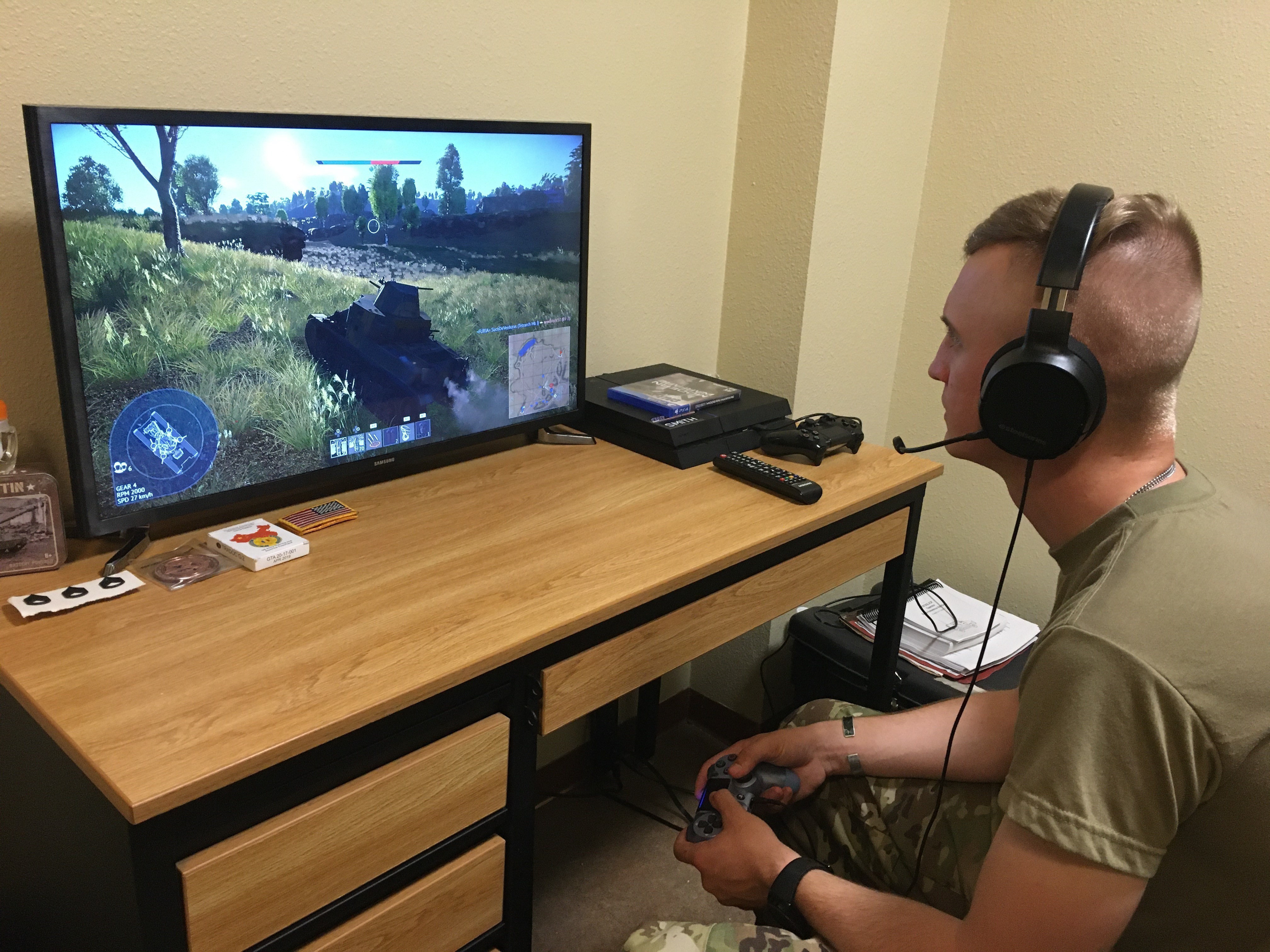In an indoor setting with beige walls, this photograph captures a soldier deeply immersed in a war-themed video game. He's seated at a modest, black-framed wooden desk, much like one found in a dormitory. The desk holds a large monitor displaying a first-person shooter game, featuring a tank in an open field of grass. To the right of the monitor sits a sleek, black video game console, alongside a matching black controller and joystick. The soldier, sporting a marine haircut and outfitted in a khaki t-shirt and desert camouflage pants, grips the controller with both hands. Donning a substantial black headset with a built-in microphone, he is intensely focused on the game.